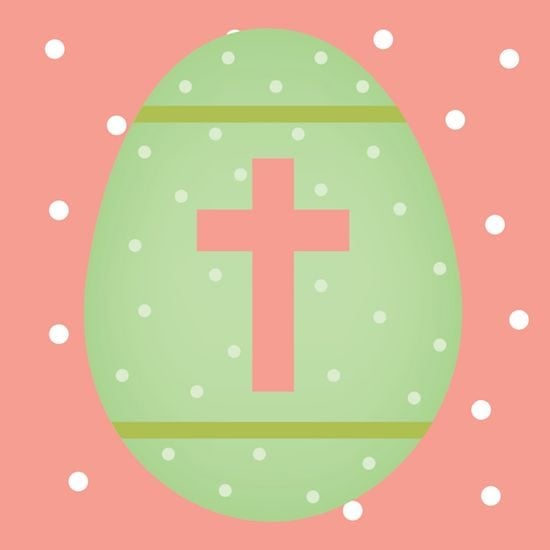The image showcases a digitally created graphic of an Easter egg. The background consists of a rose-colored square, within which sits a centrally placed, vertically oriented light green, egg-shaped area. The egg does not touch the top and bottom edges of the square, leaving ample rose-colored space around it.

On the left side of the egg, there are five large white dots forming a nearly vertical sequence: the topmost dot is in the upper left quadrant, the second dot is adjacent to the egg, and the remaining three dots descend in a line, with the final dot slightly closer to the egg. On the right side, eight large white dots are arranged: the top two dots form a triangle, two more dots near the egg, followed by four dots curving downward in a slight wave pattern, culminating in a dot attached to the bottom right of the egg.

Inside the egg, numerous smaller pale green polka dots are scattered throughout. A thick, rose-colored crucifix stands prominently in the center of the egg. Along the egg’s width, a rye grass-colored stripe runs above and another below the cross, neither touching it. The image uses colors such as pink, white, light green, lime green, and rose, and the entire composition appears to be meticulously computer-generated.